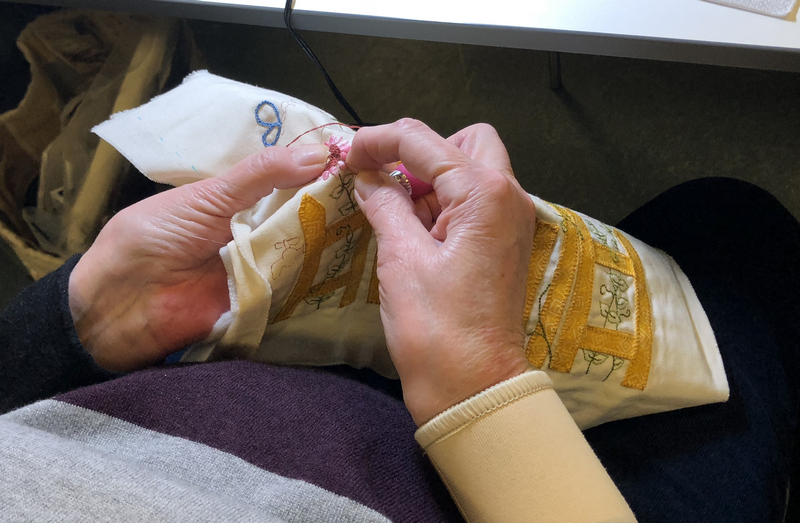In this close-up image, an elderly woman is seated and engaged in knitting or sewing. She is holding a piece of white cloth, into which she is intricately stitching a design. The design features a yellow pattern that resembles a fence and includes a pink flower under her left thumb, highlighting the delicate detail of her work. Her hands are slightly wrinkled, suggesting her advanced age. She meticulously maneuvers a needle with her right hand into the white cloth.

In the background, a white table can be partially seen, likely made of classic materials. The woman is dressed in a long-sleeve, striped shirt with varying colors: the top part is purple, the middle sections are gray, and the different sleeves are black and beige respectively. She is also wearing dark blue jeans, visible on the right side of the image. The overall scene captures the patience and skill of the woman as she works on her detailed needlecraft.